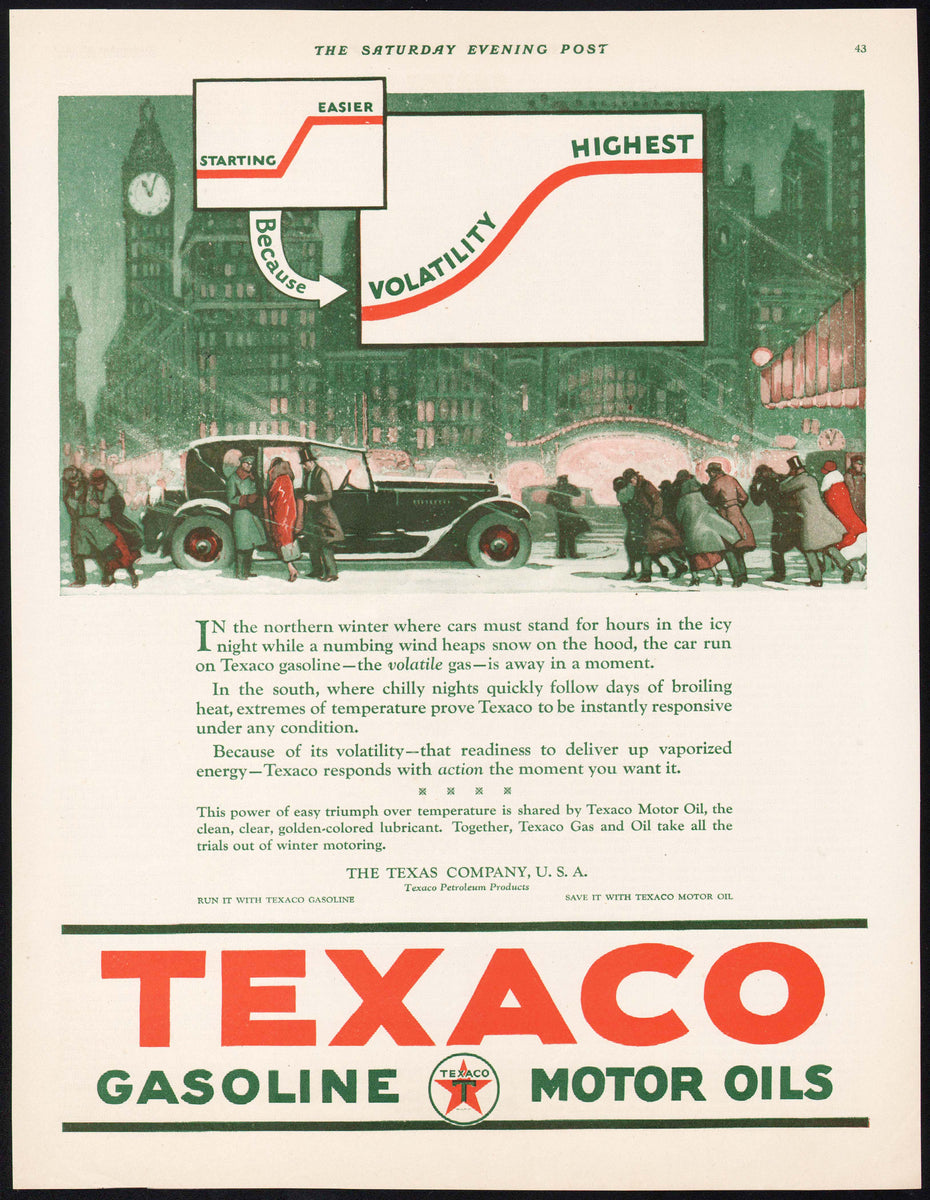This is an image of an old advertisement from the Saturday Evening Post. The poster has black borders framing an off-white background. At the top, there is a green-tinted image of a cityscape featuring a clock tower, flanked by older-style buildings. Below this, there is a detailed winter scene depicting people bundled in winter coats, walking along snow-covered streets. To the left, a vintage black car stands out prominently. 

The advertisement is split with a white square at the top featuring the text "Starting easier" in green letters, crossed by a red line. Another white square further down, also intersected by the red line, reads "Because with the highest volatility" in green letters and includes a white arrow. 

Beneath the winter scene, a few paragraphs of text describe the virtues of Texaco gasoline, particularly emphasizing its performance in extreme weather conditions. The text highlights the quick start capability of cars using Texaco gasoline in both cold northern winters and the fluctuating temperatures of the southern climate.

Finally, at the bottom of the advertisement, the name "Texaco" is boldly printed in large red letters, with "gasoline motor oils" underneath in green.